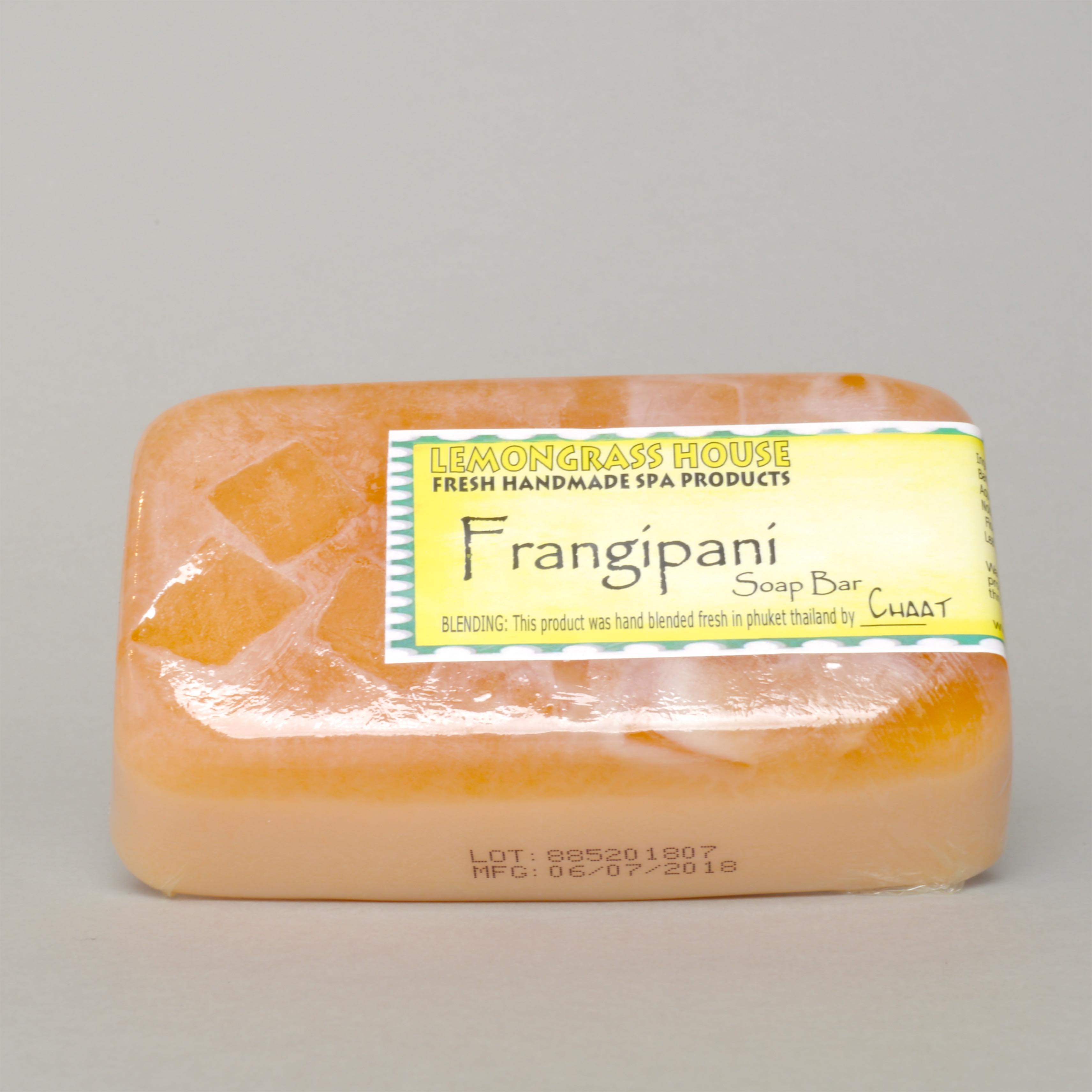This image features an orange, cuboidal soap bar delicately wrapped in transparent cellophane packaging. The soap, with a semi-transparent, sherbet-like peach hue on both its top and bottom, is prominently labeled. The label, with its eye-catching yellow color and a wavy green border, details that it’s a product from Lemongrass House, stating "Fresh Handmade Spa Products" and "Frangipani Soap Bar." Additional handwritten text informs that the soap was freshly hand-blended in Phuket, Thailand by Chhat. The manufacturing date is noted as 06/07/2018, with a lot number printed on one side. The setting features a light, beige-gray background that allows the vibrancy of the soap bar to stand out.